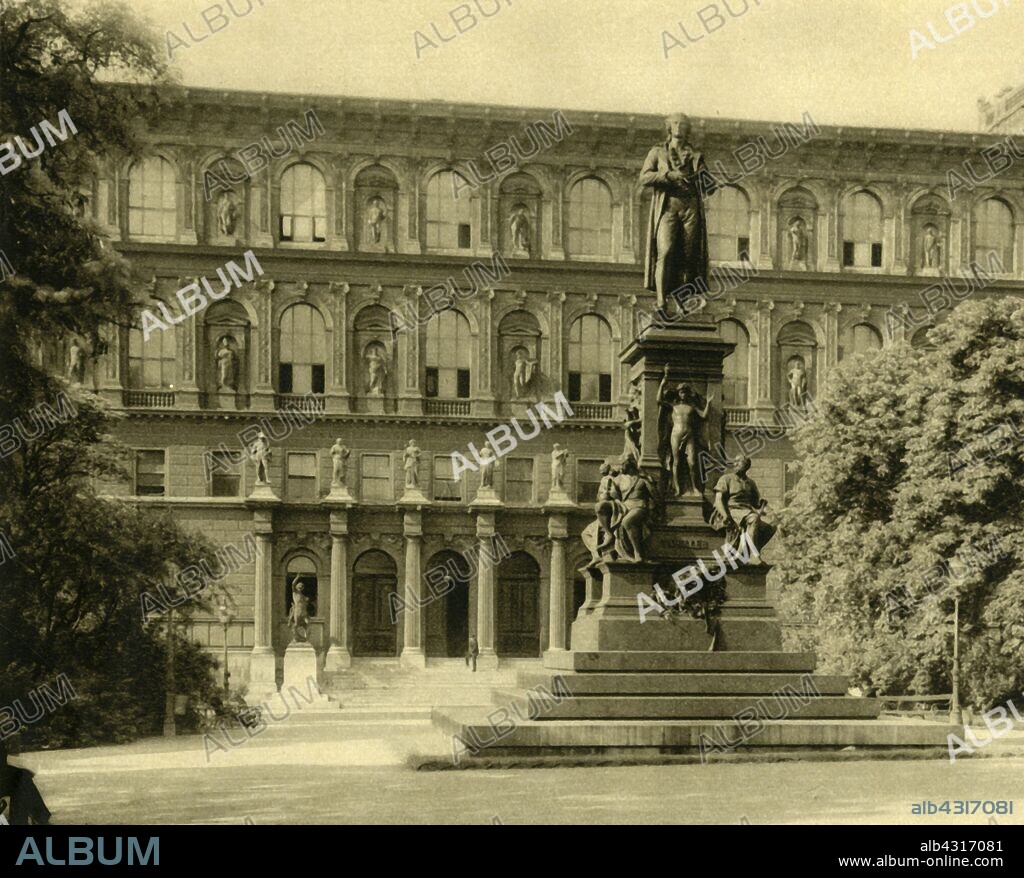This highly detailed black and white stock photo, heavily watermarked with the word "album" diagonally across the image, showcases a grand, historic building featuring multiple levels uniformly decorated with statues. The building has four floors, each adorned with statues situated in alcoves between tall windows. The façade exhibits many arches and sizable dome windows, partly obscured by large trees, including a prominent pine and another coniferous tree on either side in the foreground. 

Dominating the foreground is a monumental statue set in a grassy area in front of the building. The statue stands atop a square pedestal with five steps leading up to a figure dressed as an older English or American gentleman in a long cloak, looking upward and holding something in his arms. Surrounding him are various smaller statues, depicting children and elderly men, arranged on the steps and either side of the pedestal. 

The base of the statue, which is ensconced in front of three sets of large wooden doors—one of which is open—serves as a central focal point for the scene. The blurred statues within the building arches, coupled with the trees partially obscuring the view, lend a classical and somewhat ethereal quality to the image. A banner with the website, code details, and additional "album" watermarks appears along the bottom left and right of the image.